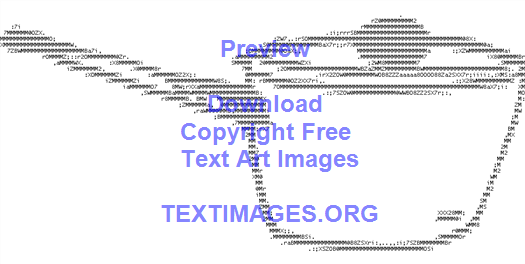The image features a pixelated gray sauce pot with a lid against a completely white background. The pot, outlined meticulously in letters and numbers, bears several inscriptions in various colors. On the lid, written in purple, is the word "preview." On the body of the pot, numerous phrases are inscribed, including "download," "copyright free," "text art images," and "textimages.org" in blue and purple blueprint style. The whole depiction appears to be a form of clip art or text art, combining words and a design in a unique graphical format.